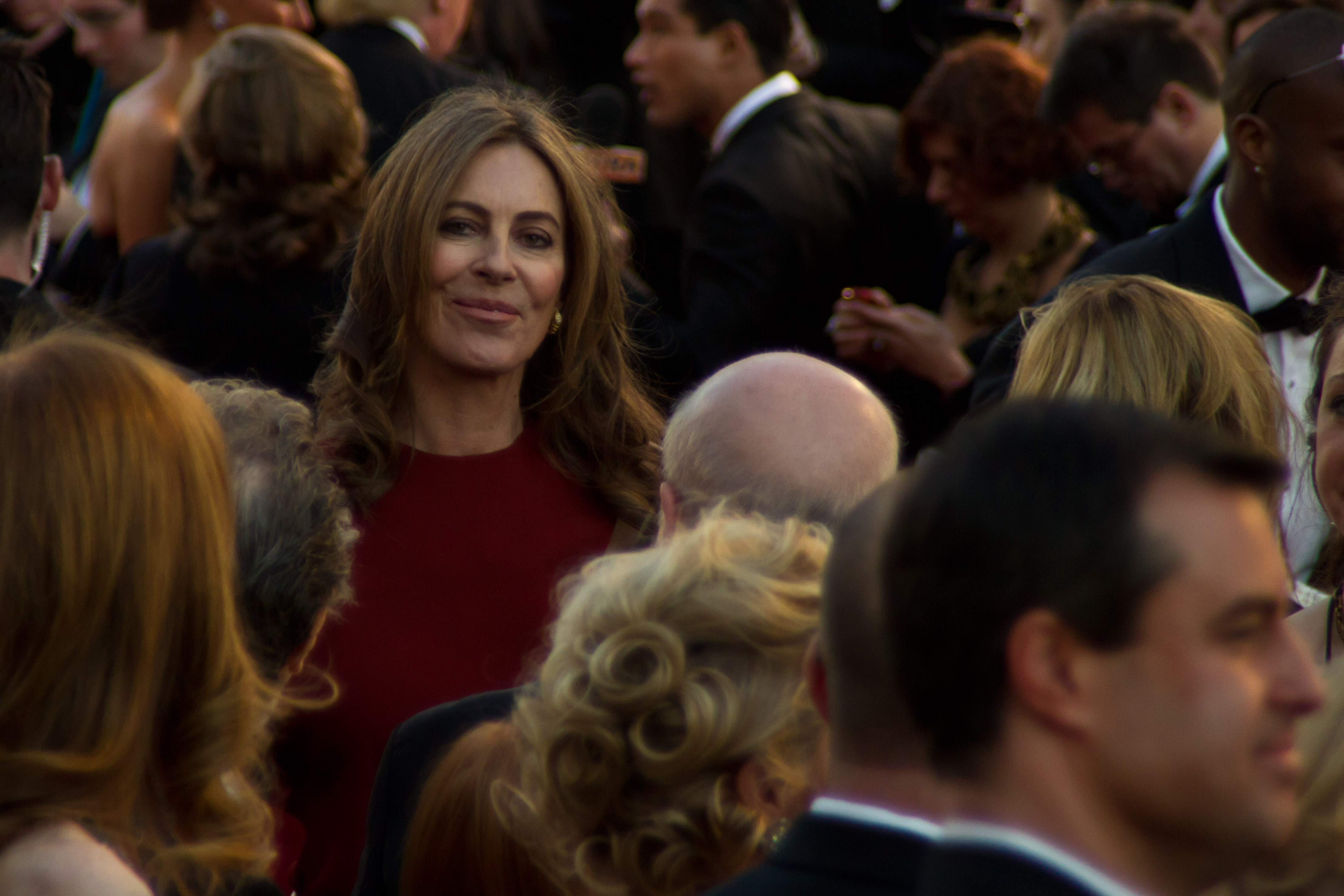The image captures a lively outdoor celebrity event, showcasing a crowd of people dressed to the nines. The main focus is a striking woman positioned slightly left of center. She commands attention with her long brunette hair, a burgundy dress or top, pink lipstick, and gold earrings. Her smirk and green eyes set her apart, as she looks directly at the camera while everyone else glances away. The bustling backdrop features men in tuxedos and women in formal attire, with one man in a black suit and white shirt, notably positioned in the bottom right corner, resembling George Clooney. Adding to the scene's sophistication, another man can be seen in the background conducting an interview with a microphone amidst a sea of elegantly dressed attendees. This setting, filled with peach, pink, red, maroon, and various shades of black and brown, hints at the presence of professional photographers or paparazzi, further indicating the event's high-profile nature.